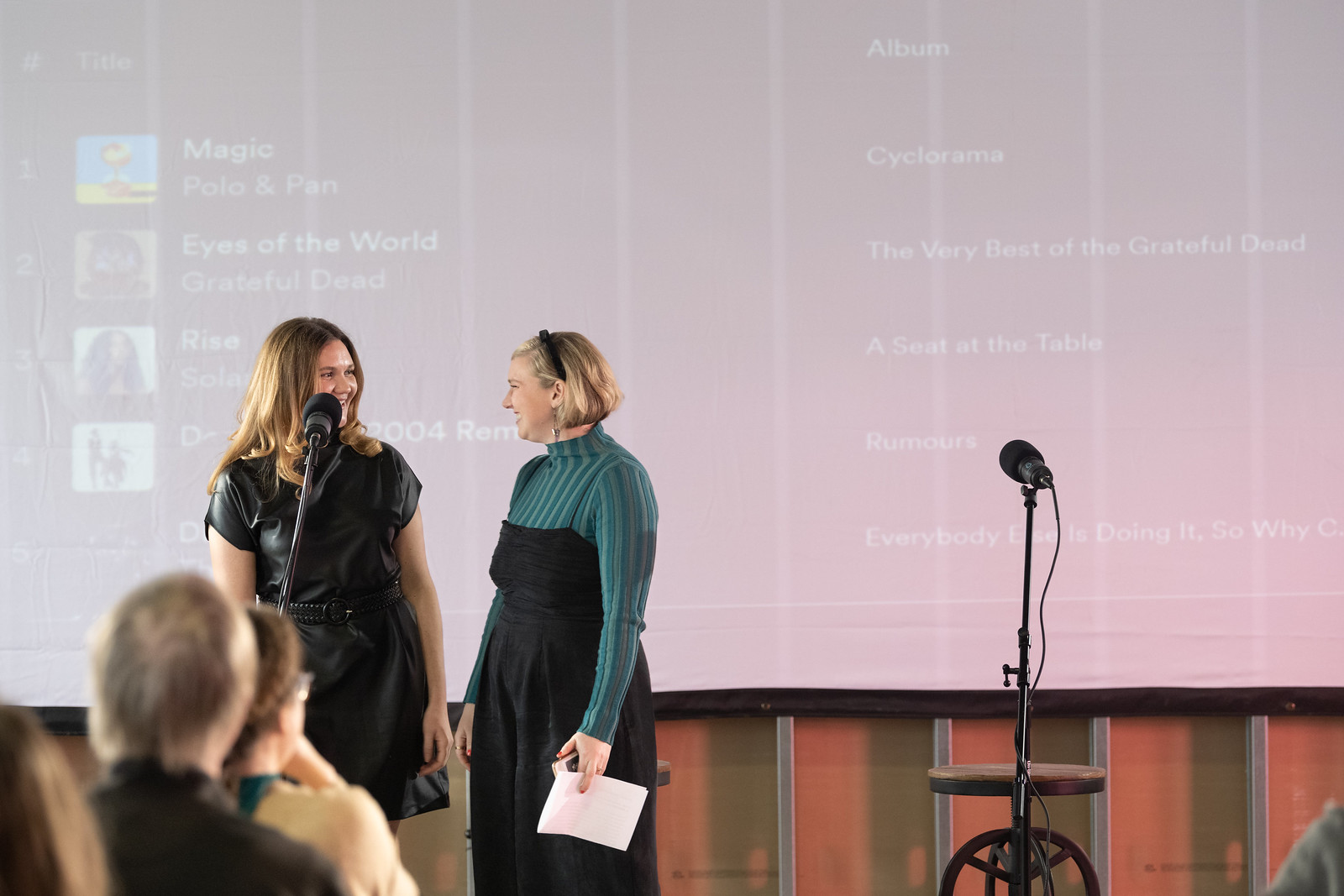The image depicts two Caucasian women on a stage in front of a projection screen, standing behind a microphone. One microphone is unattended to their right, positioned in front of an empty chair. The woman on the left, who has long, slightly wavy light brown hair, is wearing a black leather dress that is belted at the waist and falls to just above her knees. The woman to her right is dressed in a dark green turtleneck underneath a black spaghetti strap dress and holds a phone and a piece of paper. The background features a projection screen displaying a playlist with song titles and album covers, including "Magic" by Polo & Pan, "Eyes of the World" by Grateful Dead, and "Rise" by Solange, among others. Both women are speaking into a microphone and appear to be engaged with the content on the screen, looking towards each other as they do so.